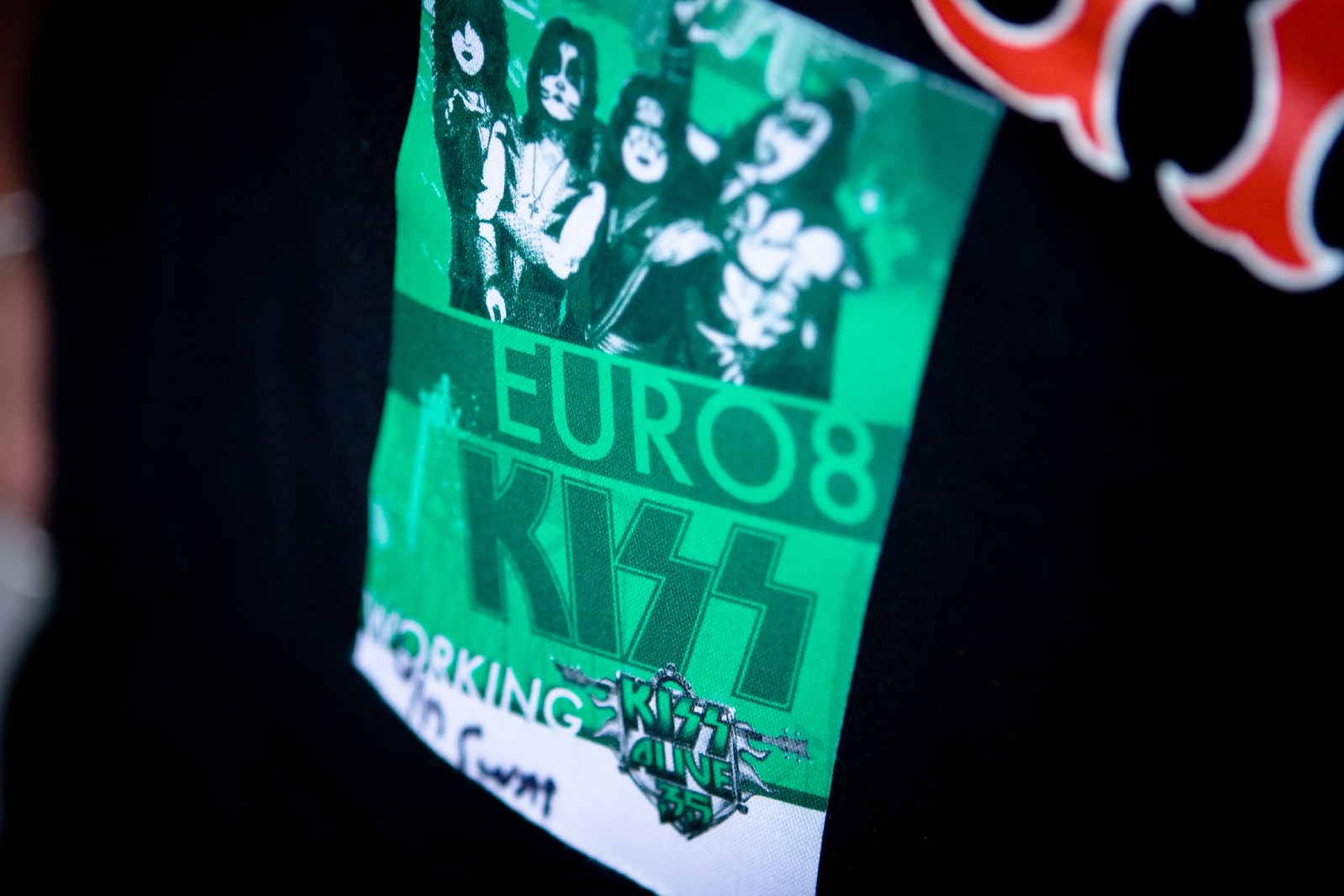This image displays a green concert badge or poster featuring the iconic rock band KISS. Positioned at the top, an image showcases the four band members—Paul Stanley, Peter Criss, Ace Frehley, and Gene Simmons—in their signature black and white makeup and costumes. Below the band members' photo, the badge reads "EURO 8" and prominently displays the KISS logo in the classic lettering style. The text beneath it includes "KISS Alive 35" and "working," signifying it’s likely for crew members involved in a European tour. The background behind the badge or poster is black, with some partially visible red letters or shapes outlined in white in the top right corner. The badge also features handwritten letters "SWA" or "SWAT" at the bottom, possibly a signature or a note. The black background and reflective green text add to the badge's visually striking appearance, making it a notable piece of concert memorabilia.